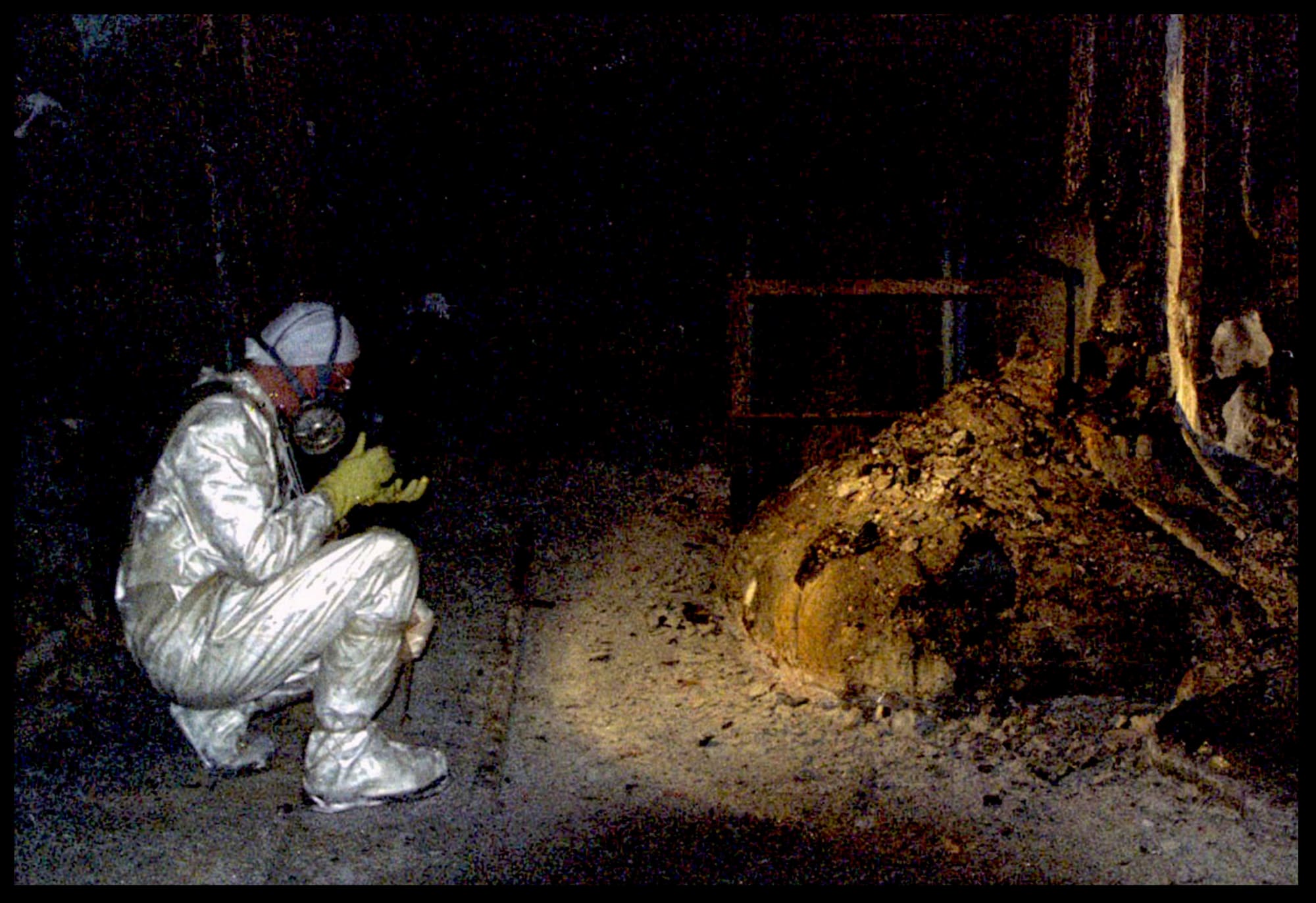This detailed photograph, captured in a darkened interior space, depicts an investigative scene, likely set at night. Dominating the left side of the image is an investigator, clad head-to-toe in a protective silver suit with yellow gloves, a respirator mask, and a head covering. The investigator is taking pictures of the scene using a camera with a light, focusing on a pile of rubble positioned to the right of the image. The area appears to be the site of severe damage, resembling the aftermath of a fire or a possibly a toxic exposure, indicated by the investigator's protective gear. The scene suggests an environment with hazardous conditions, akin to the infamous photograph taken at the Chernobyl disaster site, capturing the gravity of the damage and the meticulous efforts to document it. The photograph, in landscape orientation, uses the play of darkness and light to enhance its somber and realistic representation.